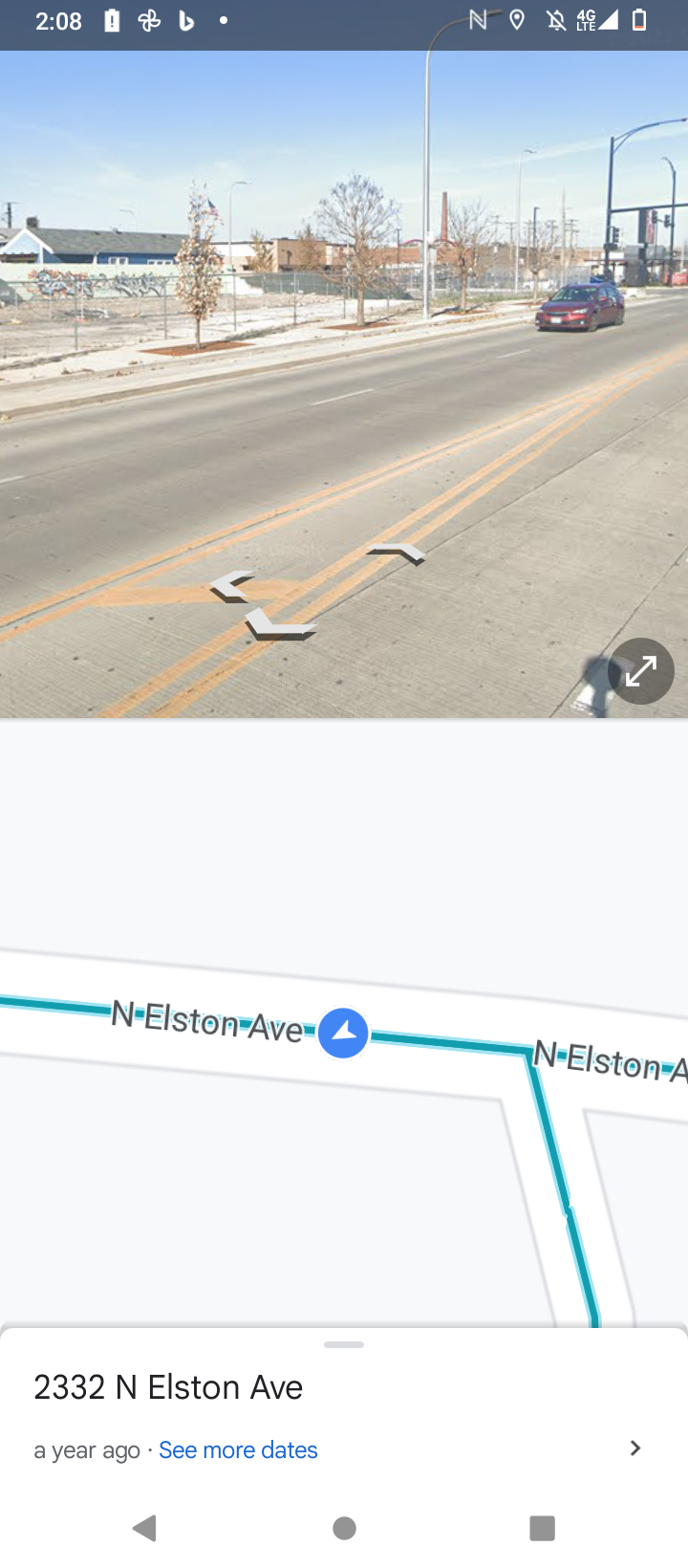This detailed screenshot image from a smartphone is divided into two sections. The upper portion showcases a street view of a road featuring a distinct double yellow line that divides the two lanes. Centered in the image, a reddish-colored car is visible in one of the lanes. The scene is notably barren, indicative of winter, as the trees lining the road are devoid of leaves. Beneath this street view section, the lower part of the screenshot displays a map segment highlighting an arrow pointing along North Elston Avenue. Complementing the arrow, a prominent green line traces the streets, suggesting a navigational route.